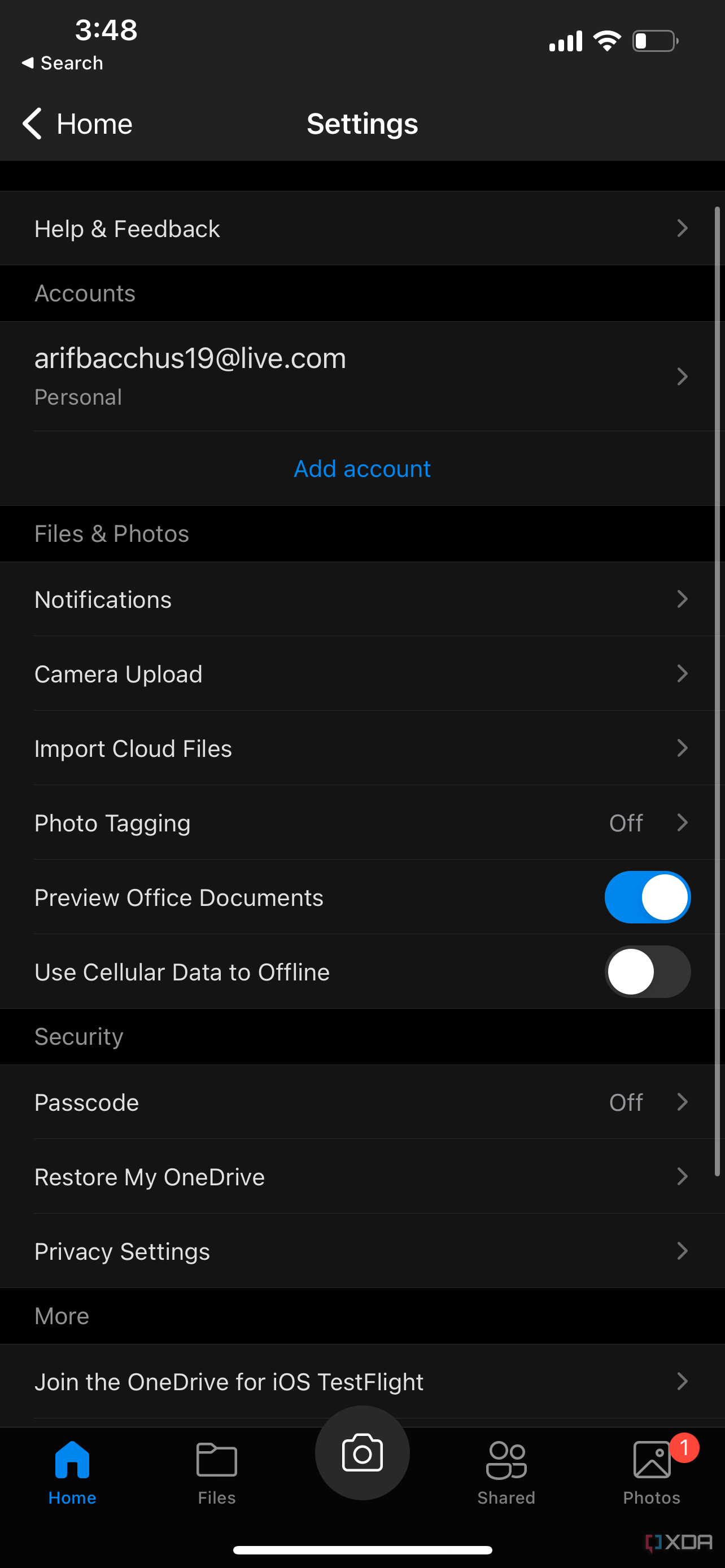This image depicts a smartphone screenshot. Detailed visual elements include the following:

- In the top right corner of the screen, a battery icon indicates a low charge, approximately 20% remaining. Adjacent to this is the Wi-Fi strength icon with full signal strength, represented by four bars. The phone’s signal strength icon, also displaying four bars, is positioned to the left of the Wi-Fi indicator.
- The top-left corner shows the current time as 3:48. Directly beneath the time, there is the word "Search" accompanied by a left-facing arrow, which resembles a white triangle on its left side.
- Centrally at the top, the word "Settings" is prominently displayed in white text.
- The main content of the screenshot starts with a single section labeled "Help & feedback" on the far left.
- The second section features two rows: the first row labeled "Accounts" with an email account listed, and the second row labeled "Personal" with an "Add account" option highlighted in blue.
- Further down, there are multiple sections with icons and labels. One section, labeled "Files and Photos," consists of six rows detailing options such as "Notifications," "Camera upload," "Import cloud files," "Photo tagging," "Preview office documents," and "Use cellular data to offline."

The screenshot provides a detailed view of various phone settings and account options, offering comprehensive insights into the phone’s current status and configurations.